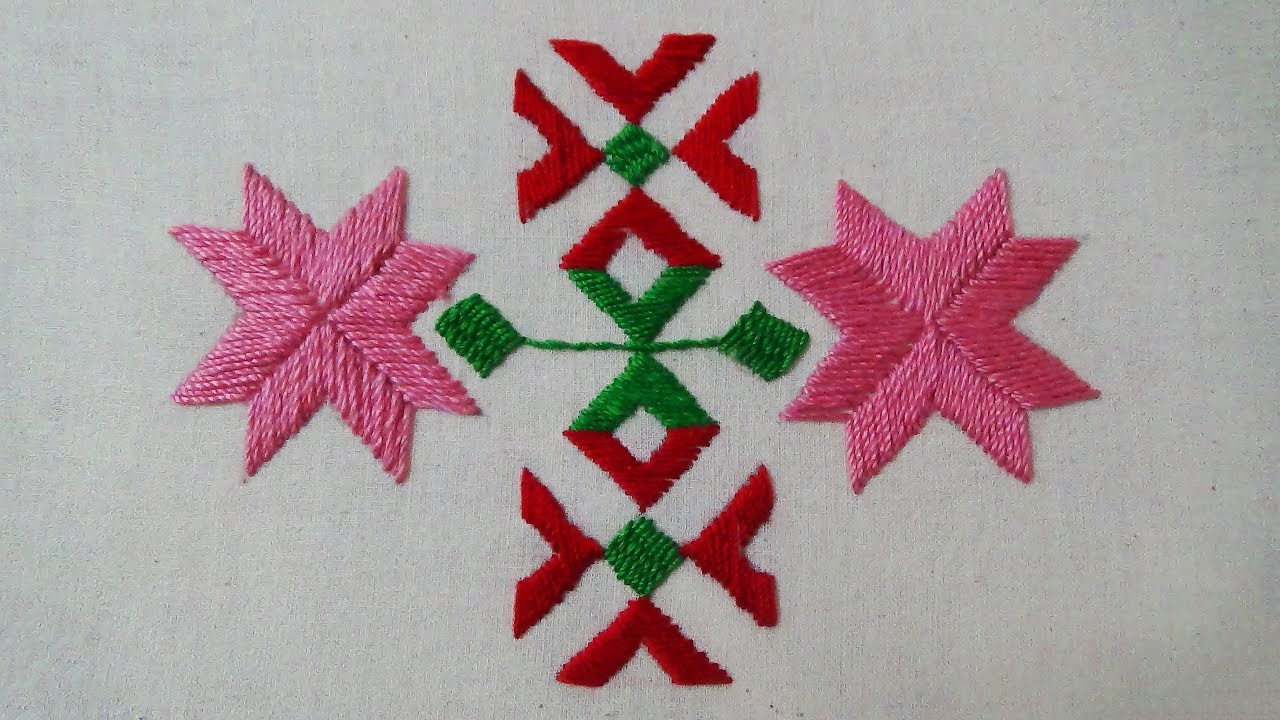This image depicts an intricate piece of embroidery on a linen-colored, perhaps white, fabric background. The embroidery features three primary colors: a dark red, a dark green, and a bright pink. Centrally, the design showcases a green X with four outward-pointing arms, intersected vertically by a symmetrical pattern of red Vs. At the core of this arrangement lies a delicate green square. Flanking this central motif are two bright pink, star-like designs—each resembling an eight-pointed star or snowflake with pairs of points spaced evenly around the shape. The repetitive symmetry and the festive color palette of dark red, dark green, and bright pink suggest a holiday or Christmas theme, reminiscent of patterns often seen on seasonal sweaters.